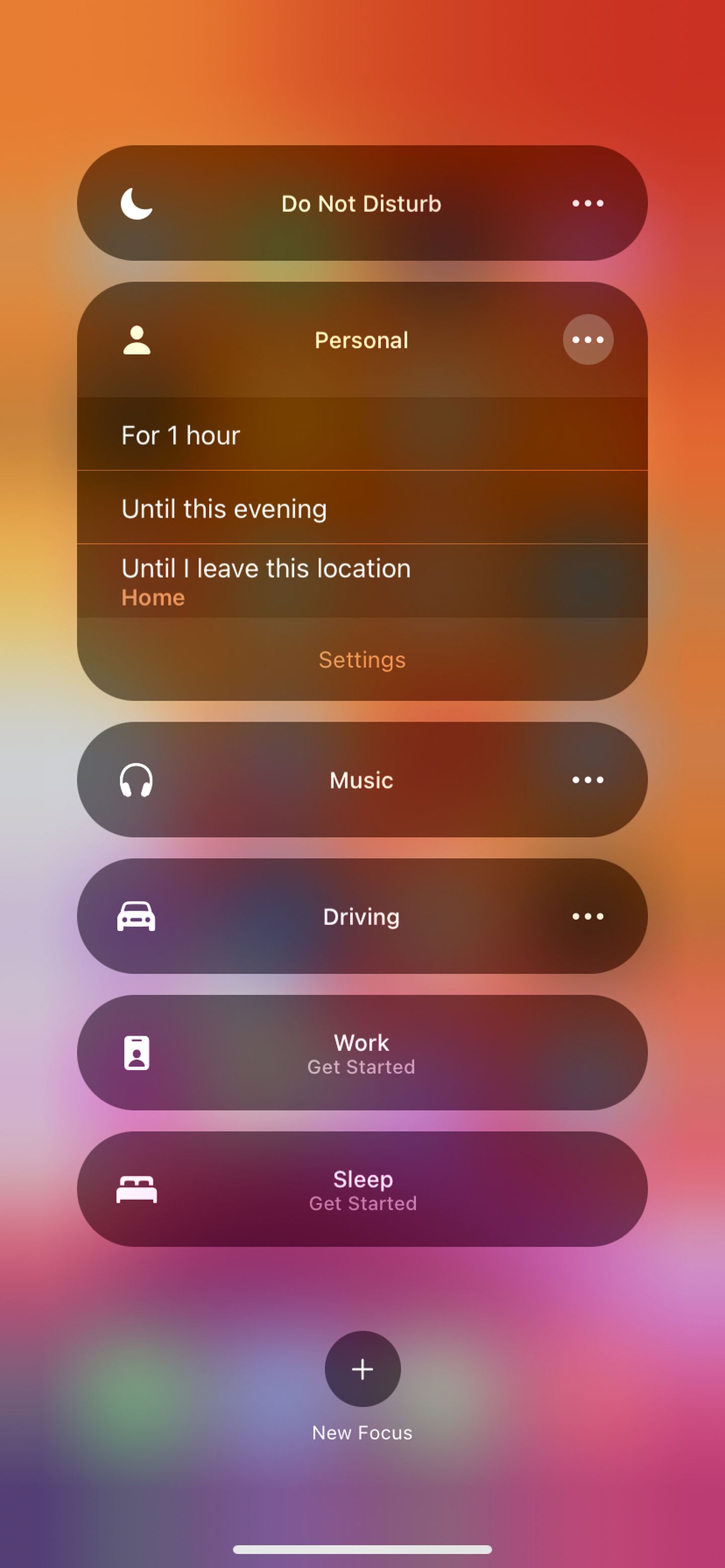The image depicts a series of overlay shortcut scenes on a home screen with a blurred background. The background transitions from pink at the bottom to orange at the top. The shortcut scenes have a transparent black backdrop.

At the top, there is a "Do Not Disturb" feature indicated by a white moon icon and text. The second scene, labeled "Personal," is currently activated and expanded, displaying options such as "For One Hour," "Until This Evening," "Until I Leave This Location," and "Home Settings." Here, "Home Settings" is in orange, while the rest of the text is white.

The third shortcut scene is labeled "Music" and features a white headphones icon on the left side. The fourth scene, labeled "Driving," includes a car icon on the left. The fifth, "Work," displays an option to "Get Started" accompanied by a work tag icon. The final shortcut scene at the bottom is titled "Sleep" with a "Get Started" prompt and a pet icon on the left side.

At the bottom of the image, there is a large white plus sign within a circle for adding another routine or focus. Below this, the text "New Focus" appears, indicating various focus options such as "Do Not Disturb," "Personal," "Music," "Driving," "Work," and "Sleep." Users can select the focus setting that best matches their current activity.